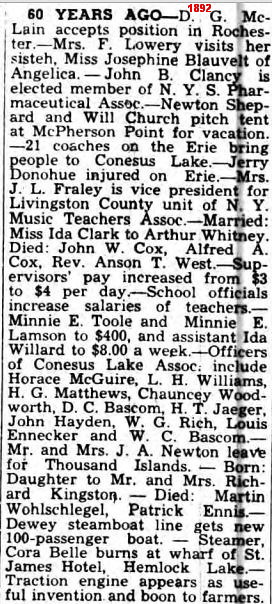The image consists of a black-and-white, one-column newspaper clipping titled "60 Years Ago." The snippet, dated 1892 in tiny red print above the title, recounts various events and personal announcements in upstate New York along the Erie Canal. Notable entries include:

- Dr. G. McLean accepting a position in Rochester.
- Mrs. F. Lowery visiting her sister, Ms. Josephine Blavet of Angelica.
- John B. Clancy being elected to the NYS Pharmacy Association.
- Newton Shepard and Will Churches pitching a tent at McPherson Point for vacation.
- 21 coaches on the Erie bringing people to Kinesis Lake.
- Jerry Donahue being injured on the Erie.

The clipping goes on to mention routine local milestones such as births and deaths, encapsulating the day-to-day life and happenings of the community decades ago. The text fills the entire image space, portraying a historical snapshot of upstate New York society.